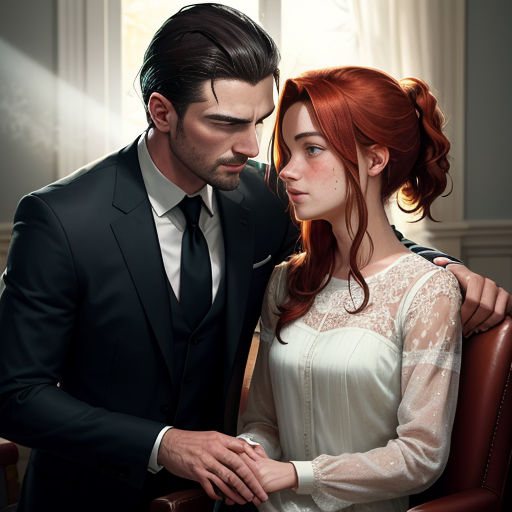The image features a man and a woman, rendered in a style that blends realism with cartoonish elements. The man, positioned on the left side of the image, is dressed in a dark blue suit with a matching tie and a white button-up shirt. He has dark hair, combed back with some bangs falling beside his face, complemented by sideburns, a beard, and a light mustache. His light skin tone adds to his distinguished appearance. With his left arm around the woman's shoulders, he also gently holds her hands with his right hand, conveying a sense of intimacy.

The woman, seated on a reddish-brown leather chair on the right side, has a delicate frame. She wears a white, gauzy dress with lace details at the top and long sleeves. Her light skin features freckles and rosy cheeks, while her red hair is styled with bangs that frame her face, curling towards her chest, and the rest is pulled back. She gazes off into the distance, creating a serene and contemplative mood.
  
The setting of the image appears to be a softly lit room with light blue walls and white window trim. Sunlight streams in through a window behind them, illuminating the couple in a warm, gentle glow, while the rest of the room remains dimly lit.